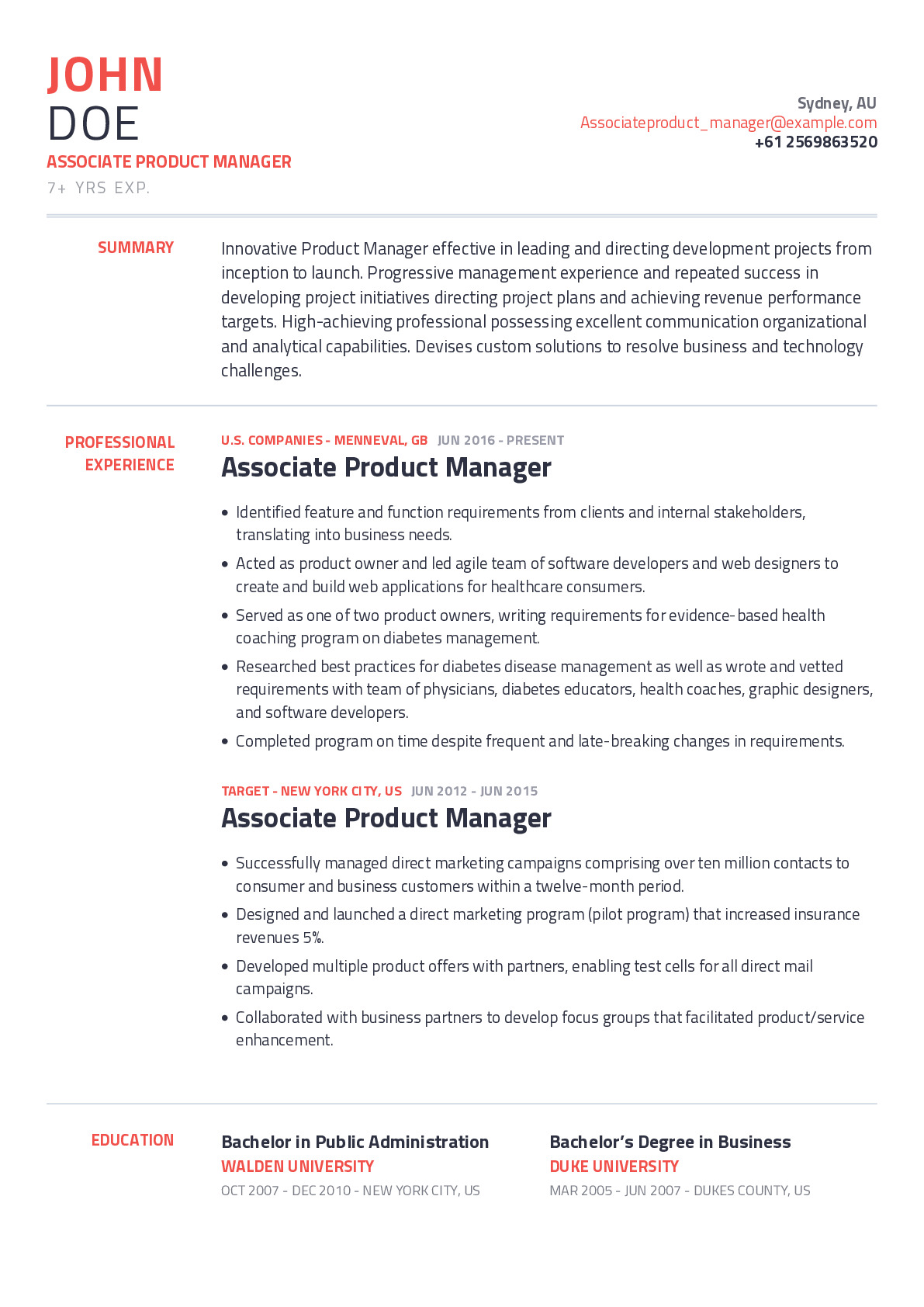The image is a detailed resume for John Doe, an Associate Product Manager with over seven years of experience. At the top left corner, his name is prominently displayed with John in red and Doe in black, followed by his title and years of experience. Adjacent to this, on the right side, is his contact information, including a phone number formatted as +61 2 5698 6352, and his professional email at example.com, located in Sydney A.U.

The resume is divided into three main sections, each separated by thin gray lines. The first section is a "Summary" highlighted in red letters, providing an insightful overview of his career. The summary states that John Doe is an innovative Product Manager with a proven track record in leading projects from inception to launch. It emphasizes his progressive management experience, successful project initiatives, ability to meet revenue performance targets, and his excellent communication, organizational, and analytical skills.

The second section, "Professional Experience," written in red, details his work history. It includes his current position at Manevel G.V., U.S. Companies, from June 2016 to the present. His role as an Associate Project Manager is documented in larger dark lettering. Accompanying this are bullet points outlining his responsibilities, such as identifying feature requirements from stakeholders, leading an agile team for healthcare web applications, and effectively managing projects to completion despite changing requirements. His previous role at Target, New York City, from June 2012 to June 2015, is similarly detailed. Key achievements include managing extensive marketing campaigns, launching pilot programs, and developing product offers and focus groups that enhanced service offerings.

The final section, "Education," written in red, lists his academic credentials. John Doe holds a Bachelor's Degree in Public Administration from Walden University and a Bachelor's Degree in Business from Duke University. The corresponding dates and locations of his education span from October 2007 to December 2010 in New York City and from March 2005 to June 2007 in Dukes County, U.S.

This comprehensive resume blends professional experience, educational background, and personal summary into a clear and structured format, presenting John Doe as a highly qualified candidate for a Product Manager role.